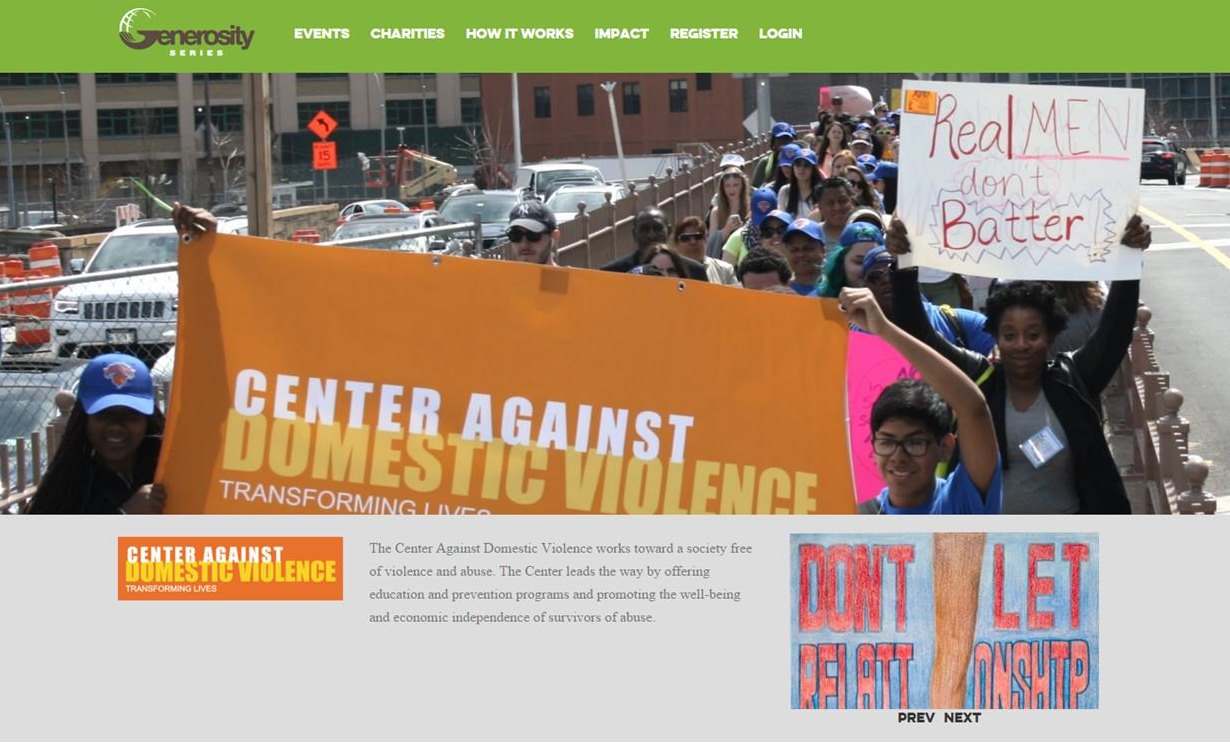This is the homepage of a website with a prominent theme focusing on generosity. At the top, there's a green banner with the word "Generosity" in brown and "Series" in white. The navigation bar features links in white text, including "Events," "Charities," "How It Works," "Impact," "Register," and "Login."

Spanning the width of the page, there's a large, impactful photograph of people marching in support of a cause. Among the marchers, one person is holding a yellow-orange poster with white and orange text that reads "Center Against Domestic Violence." Another individual is displaying a handmade sign in white with the message "Real Men Don’t Batter."

Below the photograph, a gray bar highlights the mission statement of the Center Against Domestic Violence. It states, "Transforming lives: The Center Against Domestic Violence works towards a society free of violence and abuse. The Center leads the way by offering education and prevention programs and promoting the well-being and economic independence of survivors of abuse."

Additionally, there is an eye-catching poster with a somewhat ambiguous message about relationships and violence, partially readable as "Don't let ... on ship relationship."

The overall aesthetic of the page combines advocacy, community engagement, and a firm commitment to ending domestic violence through comprehensive support and educational initiatives.